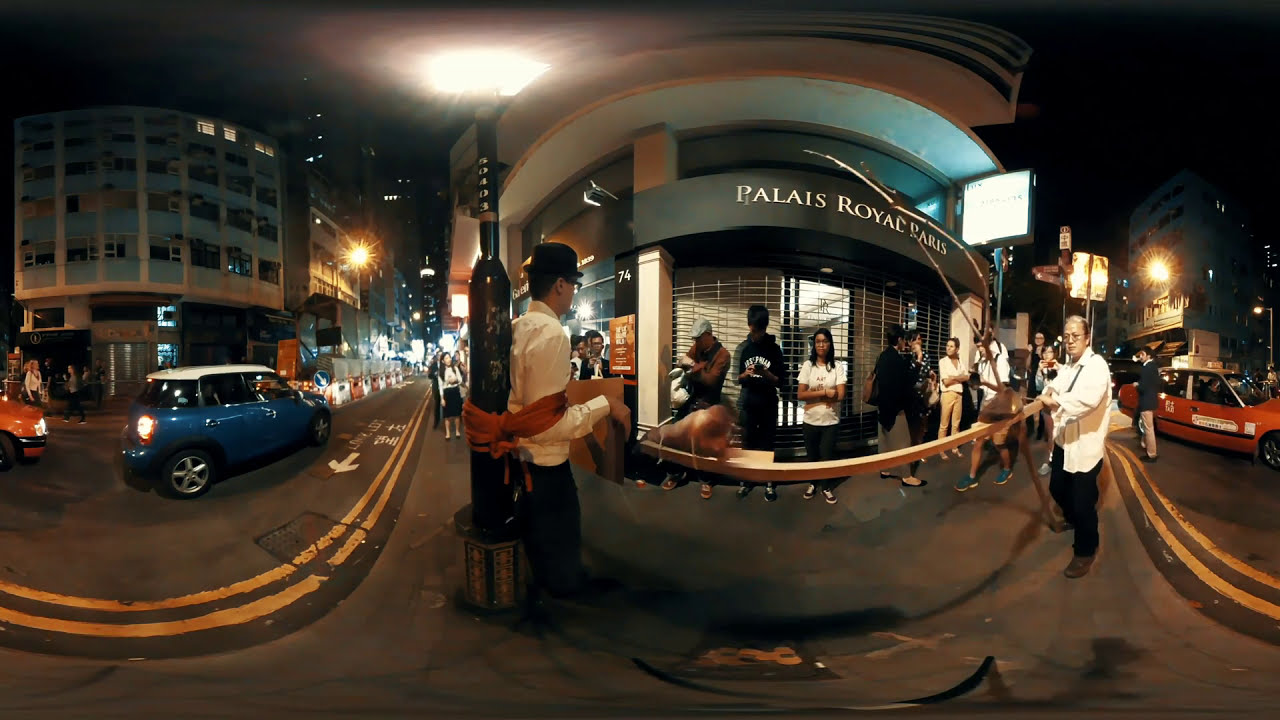In this detailed image, a bustling street scene outside the Palais Royal in Paris is captured, possibly through a virtual reality lens giving it a slightly wavy and 3D appearance. A diverse crowd of men and women, indicative of the city's vibrant public life, gathers around a significant booth that clearly displays the words "Palais Royal Paris" in bold white letters. The scene is set against a backdrop featuring buildings and a busy street marked with yellow lines. Notably, a yellow car and a blue car are parked nearby, enhancing the sense of a lively urban environment. Central to the image is a young man making a statement by being chained with red rope to a light pole at the edge of a sidewalk that seems to form a U-turn. This individual draws considerable attention from the passersby. He is distinctively dressed in a white long-sleeved business shirt, a black derby hat, and black horn-rimmed plastic eyeglasses. The streets are marked with pylons indicating a detour, adding to the sense of a busy, dynamic location. The entire scene reflects the lively, multifaceted character of this Parisian locale.